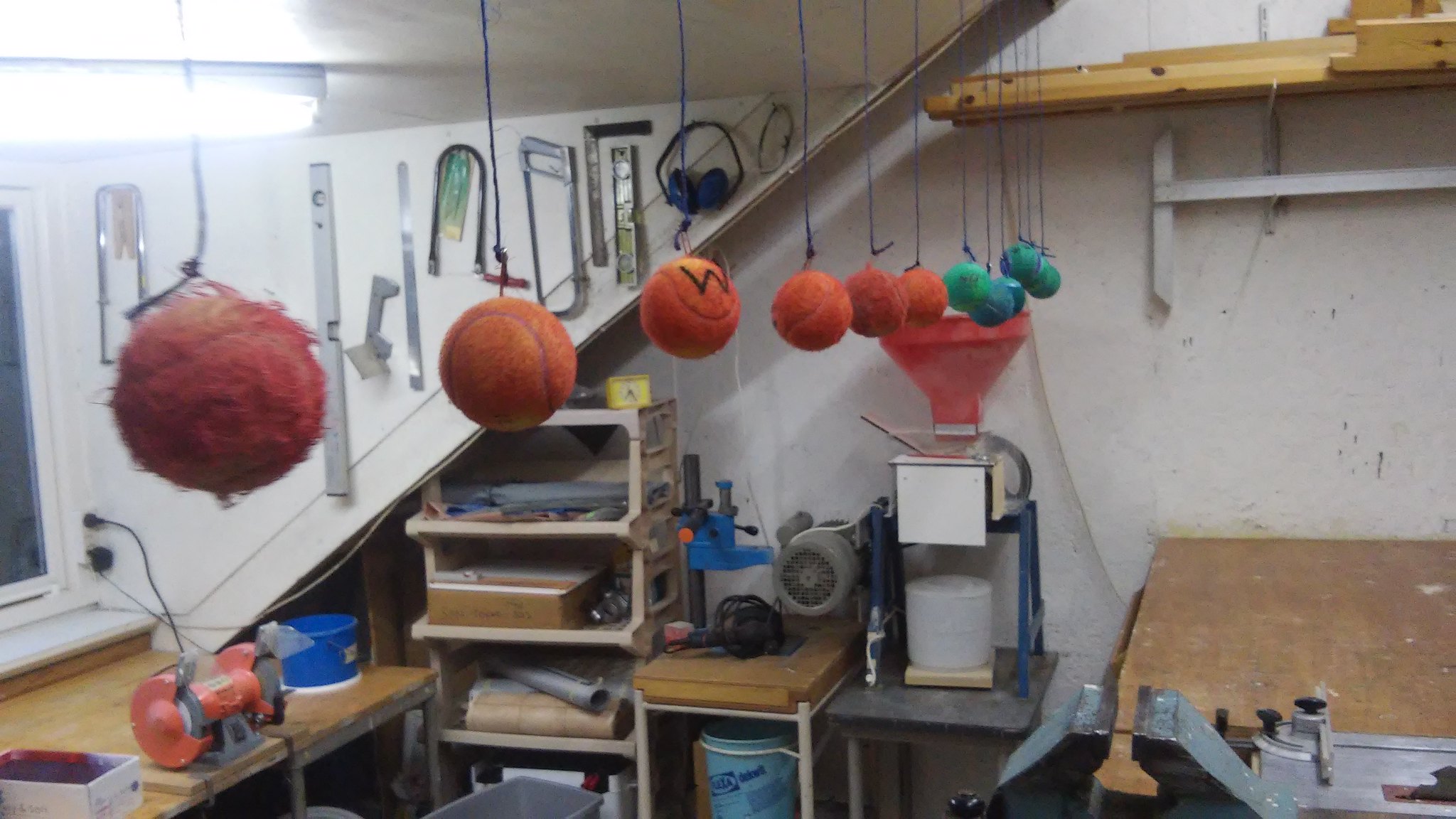The image depicts a cluttered basement workshop or garage filled with various tools and equipment, suggesting a working man's DIY space. Prominently, there are different colored tennis balls—red, orange, and blue—hanging in a line from blue strings attached to the ceiling, with some showing signs of wear. Tools and measuring equipment, including saws, a level, rulers, and chainsaws, are neatly hung on the wall. An orange cutter blade machine is visible on a table, with other machines scattered around. The right side of the image features a wooden workbench with a clamp, a bucket underneath, and a woodpile stored on metal racks. The workshop is well-lit by a fluorescent light on the ceiling, and sound-canceling earmuffs hang from the wall, emphasizing a space designed for serious, potentially loud projects. There appears to be a stairway or a sloping board in the back of the image, adding to the utilitarian feel of the space.